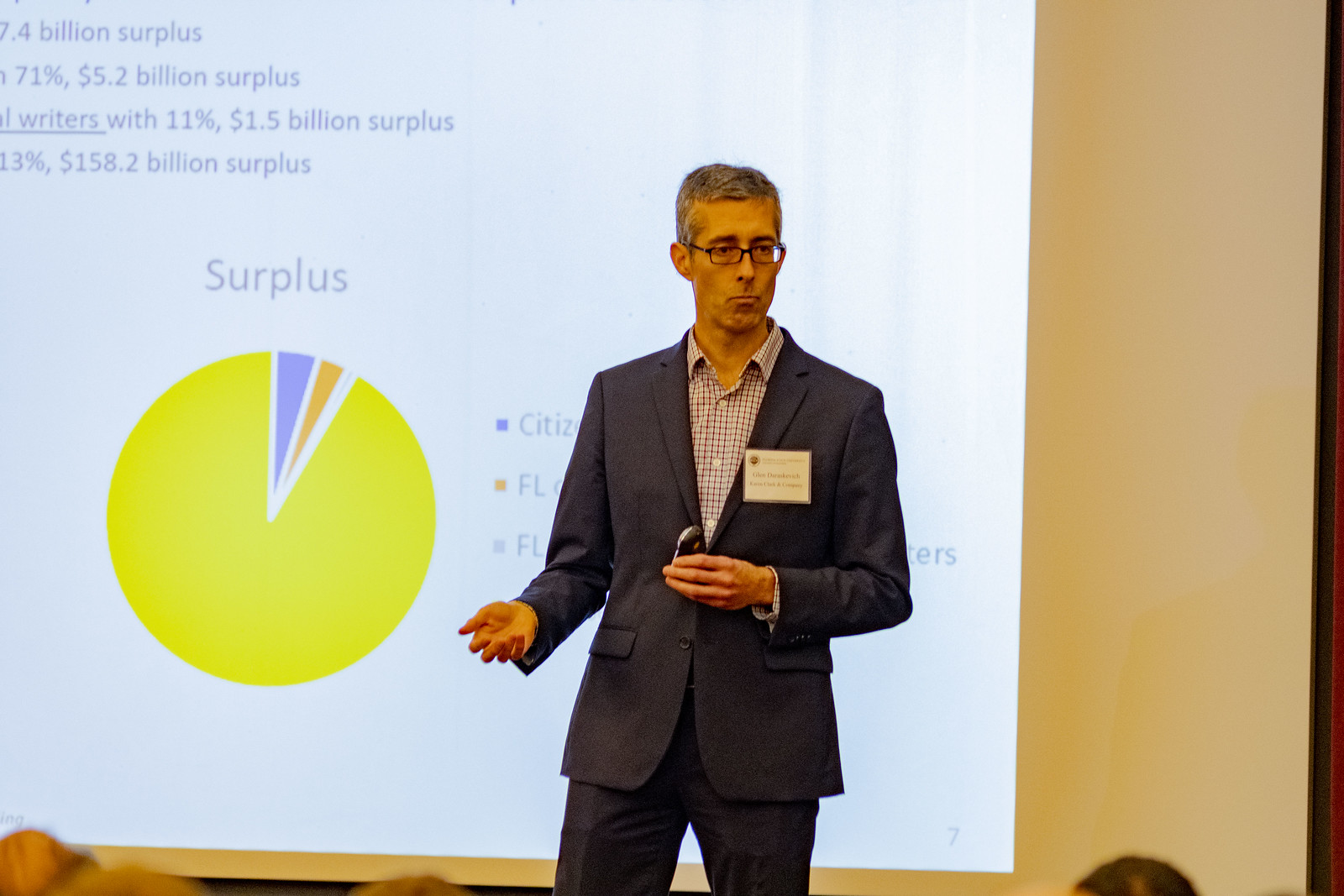In the image, a man in business casual attire, with short gray hair and rectangular glasses, stands at the center of an indoor, dimly lit room, giving a presentation. He is dressed in a dark gray suit jacket over an open-collared plaid shirt, matching dark gray pants, and holds a clicker in his left hand while gesturing with his right. The man maintains a sober expression as he addresses the audience, whose heads are partially visible at the bottom edge of the frame. Behind him, a projected image on an off-white wall displays a colorful pie chart and various financial figures. The prominent text reads "surplus," and includes detailed numbers such as "7.4 billion surplus," "71%," "5.2 billion dollar surplus," "11%," and "1.5 billion dollar surplus." The colors on the chart are black, white, yellow, purple, orange, gray, and tan, consistent with the business-like theme of the presentation at what appears to be a trade conference or similar event.